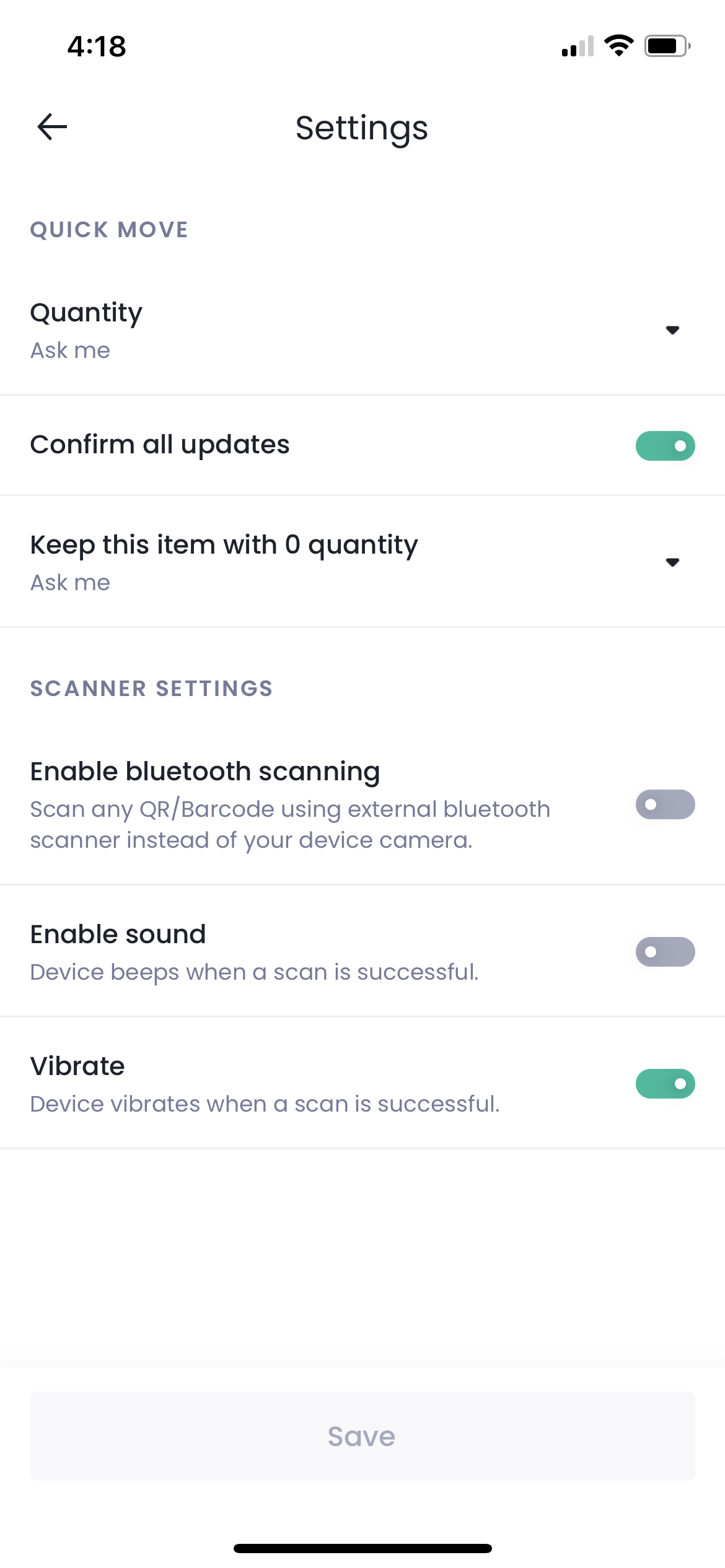Screenshot of a Phone Settings Page

The screenshot captures the settings interface of a phone's user interface. At the top, there is a navigation bar with a back arrow positioned to the left. Below this, the screen is divided into two main sections: "Quick Move" and "Scanner Settings."

In the "Quick Move" section, there are three options:
1. Quantity (featuring a down triangle icon on top).
2. Confirm All Updates (this option has a green toggle button indicating it is enabled).
3. Keep This Item with Zero Quantity (also with a down triangle icon below).

The "Scanner Settings" section contains three options:
1. Enable Bluetooth Scanning (this option is toggled off and appears in grey).
2. Enable Sound (also toggled off and grey).
3. Vibrate (toggled on and highlighted in green).

At the bottom of the screen, there is a light grey "Save" button. A black bar runs horizontally across the middle of the bottom of the screen, possibly indicating additional navigational or interface elements.